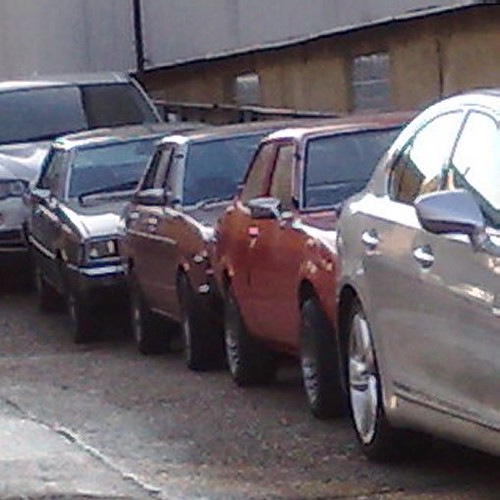This slightly blurry, grainy photograph appears to have been taken with an older camera and depicts five cars parallel parked in a line on a gray asphalt road. The cars, positioned at a slight diagonal from the camera's perspective, are set against the backdrop of a yellow building with clear square windows, which has a larger gray wall extending to the top of the image.

Starting from the right, the closest car is a silver or tan vehicle with black wheels and silver rims. Directly behind it are two glossy red cars, each with black wheels. Moving further back is a nondescript brownish-red car, also with black wheels. The final vehicle at the far end is a white SUV, which is the largest among them. The three middle cars are noticeably shorter in height than the vehicles on either edge. Notably, you can see through the dark front windshields of all five cars, and none of them appear to be occupied.